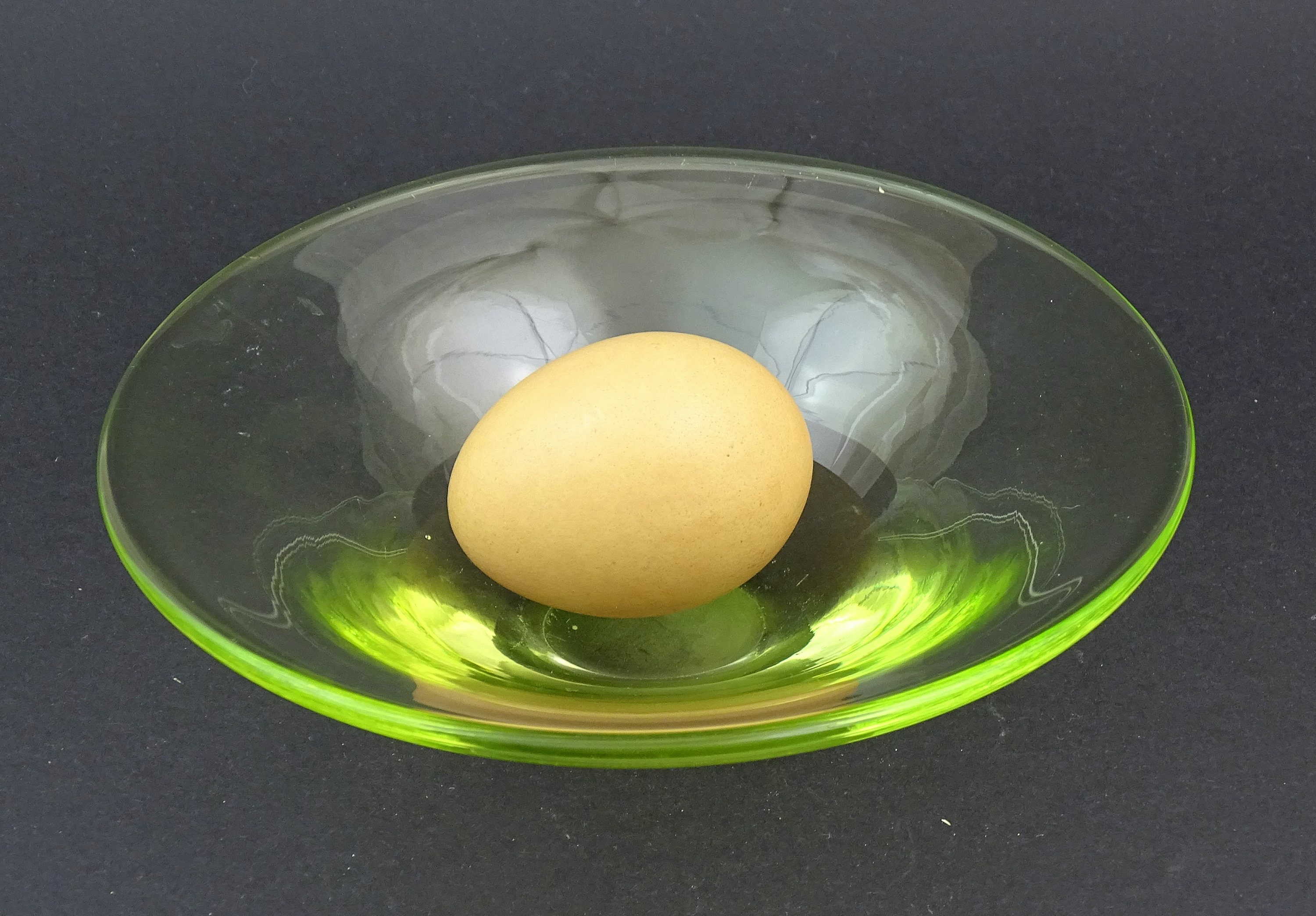This is a color photograph featuring a single light brown, oval-shaped egg, positioned centrally with its pointed side facing left. The egg rests within a glass bowl exhibiting a greenish hue, created either by the material of the bowl or lighting effects. The bowl, not completely flat, flares upwards around the edges and showcases intricate swirls of green and lime green throughout. Additionally, there are indistinct white areas in the glass, and some swirling colors of green and yellow likely caused by overhead lighting. The background is a strikingly dark brown, nearly black, which contrasts sharply with the bright bowl and egg, contributing to the photograph's artistic and dramatic presentation.